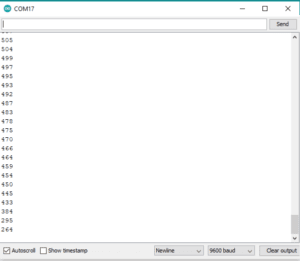The image displays a blurry screen interface. On the upper left, there is a green circle next to the label "COM1" in gray letters, followed by a question mark. Moving right across the top of the screen, there is a dash, a square, and an "X" icon. Below these controls, there is an input box for entering text, adjacent to a gray button labeled "Send".

The left side of the screen is lined with a vertical list of numbers: 305, 304, 499, 497, 495, 493, 492, 487, 483, 470, 475, 472, 466, 464, 459, 454, 450, 445, 433, 384, 295, and 264. 

At the bottom of the interface, there is a checked box labeled "Auto Sort" and an unchecked box labeled "Show Timestamp". Just below these options, there are the labels "9600 BAUD" and "Clear Output".